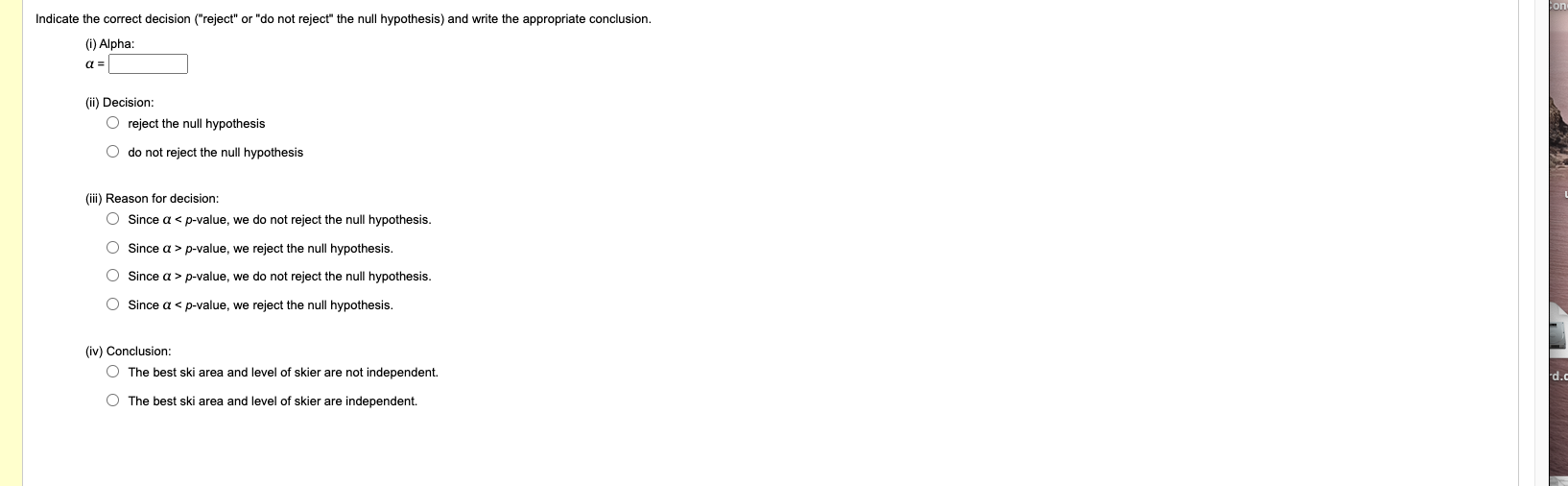The image depicts a section of a website or possibly a PDF document with a white background and a very slim yellow margin running vertically along the left edge. This margin occupies less than 10% of the entire screenshot. Within the white field of the document, black text describes various instructions and input options.

At the top, there's a heading that reads, "Indicate the correct decision (reject or do not reject the null hypothesis) and write the appropriate conclusion." Below this prompt, the word "Alpha:" appears, followed by an open text box for user input.

Further down, there is text that says "Decision:" The image then shows two radio buttons with the options: "Reject the null hypothesis" and "Do not reject the null hypothesis."

Below this, there is another prompt that appears to be related to the reason for the decision, although the exact wording is indiscernible. This section offers four possible toggle selections, though their labels are too small to read clearly.

Lastly, there is a section labeled "Conclusion:" with two toggle possibilities, again with text too small to identify.